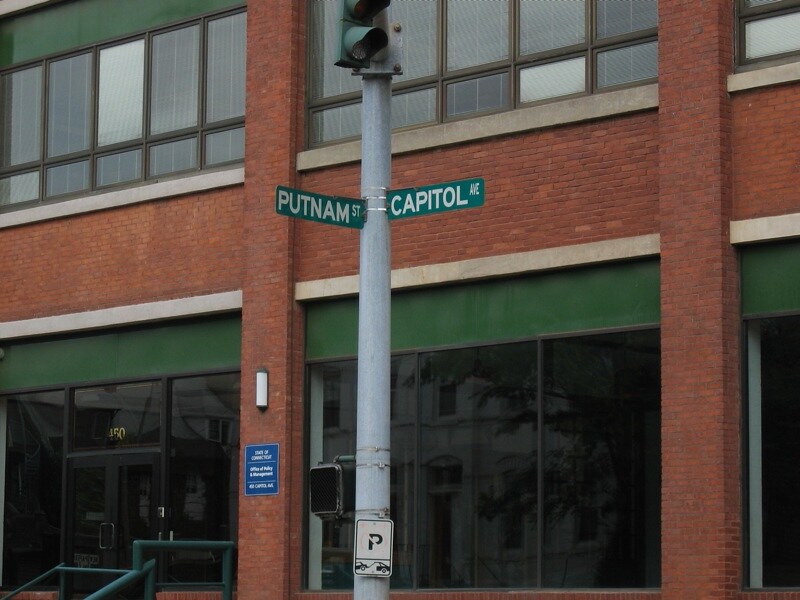This outdoor photograph showcases a two-story commercial building with a semi-modern aesthetic. The structure, constructed from red brick, features prominent large open windows on the main floor, each topped with decorative green brackets. The second story also sports smaller windows with similar green brackets, and white Venetian blinds are clearly visible behind these windows. A gold address number, 450, is displayed above the building's entrance.

In the foreground stands a green street sign with white lettering indicating the intersection of Putnam Street and Capitol Avenue. Just above this sign, a streetlight is visible, and below it, a black and white no-parking sign depicts a tow truck towing a car.

Reflections in the main floor windows reveal an older white building, some trees, and what appears to be a nearby residential building, providing a glimpse into the surrounding neighborhood.